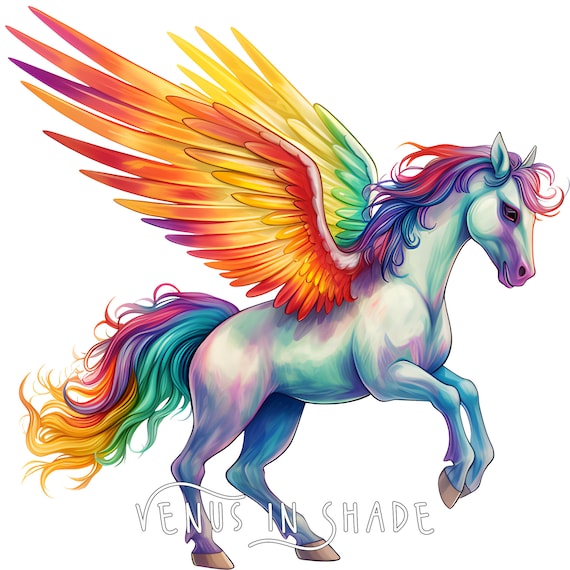This colorful illustration depicts a stylized winged horse, reminiscent of the mythical Pegasus, standing on its hind legs with its front legs raised. The horse is mainly a blend of purple, turquoise, and cream hues, with light brown hooves. Its mane and tail are an exuberant cascade of rainbow colors—red, purple, blue, pink, green, yellow, and orange—curly and flowing. The wings, which are extended upwards and out, also follow this vibrant rainbow pattern. The wing closest to the viewer showcases a gradient of orange, yellow, and purple on the underside, while the far wing displays green and yellow on the backside. The horse's ears are perky white, its eye and nostril are dark, and it has a light pink mouth. Additionally, a small mix of purple and green streaks can be seen on its body, which gives it a whimsical, multicolored appearance. At the bottom of the image, the words "Venus in shade" are inscribed with decorative swirls on the letter V and the letter S, enhancing the fantastical feel of the artwork.